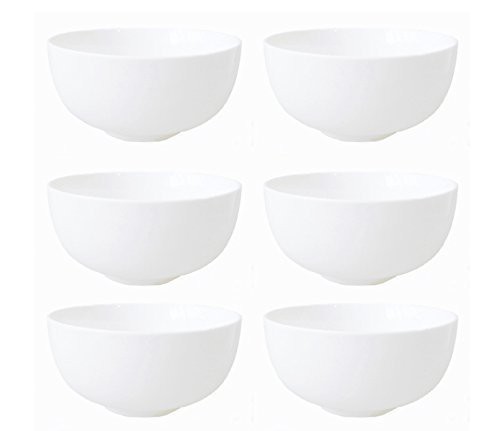This image displays a set of six identical white bowls, likely suited for soup or cereal, arranged against a solid white background. The bowls are organized in three rows, each row containing two bowls. The bowls exhibit a slight shine, indicating they might be dishwasher and microwave safe. Each bowl appears somewhat deep with a slightly raised bottom, giving the impression they’re not entirely flat on a surface. The bowls have a rounded design with a subtle shadow on their left side, enhancing their three-dimensional look. The left side of the arrangement appears slightly less bright compared to the right side, possibly due to lighting effects. Overall, the bowls are plain, functional, and uniform in appearance.